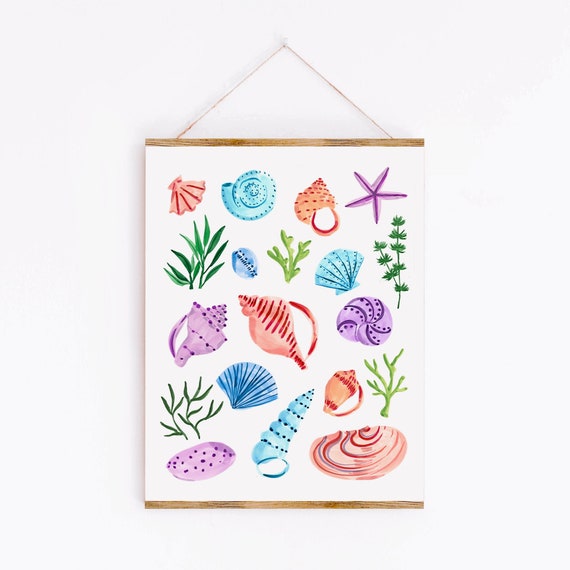The image showcases a vibrant wall banner hanging from a small red string attached at the top, displaying an array of colorful oceanic illustrations. Encased in a wooden frame with brown borders at the top and bottom, the banner features various seashells and marine life against a white background. Detailed drawings include a purple starfish, a blue clam, and a pink conch shell, as well as a purple mollusk and some small pink fish. Different marine plants, such as seaweed and green corals, are interspersed among the shells, creating a rich tapestry of underwater flora and fauna. The banner hangs perfectly straight against the wall, contributing to its visually appealing composition.